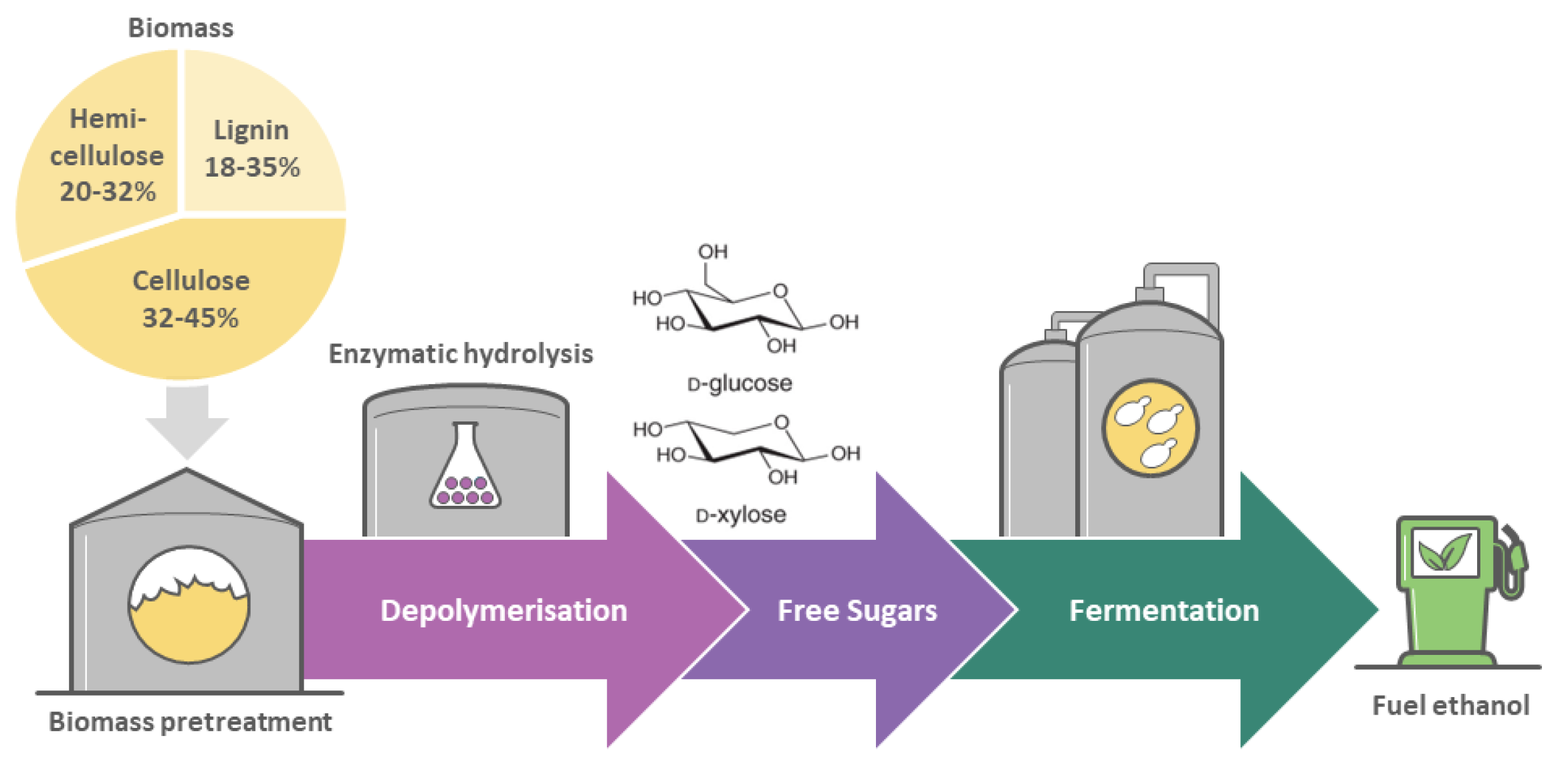This detailed infographic illustrates the multi-step process of converting biomass into ethanol fuel. Positioned on a white background, the diagram starts on the top left with a section labeled "Biomass" in black text accompanied by a pie chart shaded in various yellows. The chart quantifies the biomass composition: hemicellulose (20-32%), lignin (18-35%), and cellulose (32-45%). 

A small gray arrow points downward to a dark gray, square-shaped container with a triangular top, housing a circle that's white on the top half and yellow on the bottom, labeled "Biomass Pretreatment." 

To the right, a large purple arrow marked "Depolymerization" leads to a gray container. Within this container is a white beaker dotted with purple spots, denoting the "Enzymatic Hydrolysis" stage. This structure then transitions to smaller, detailed labels like "Free Sugars," listing components such as D-xylose and D-glucose.

Progressing further, an intermediate "Fermentation" step is depicted, showing a vat where these free sugars are processed. The final outcome is visually connected to a gas station pump icon, labeled "Fuel Ethanol," signifying the conclusion of the ethanol production process. Throughout, the infographic uses diverse visual elements to clearly delineate each stage from biomass to the production of fuel ethanol.